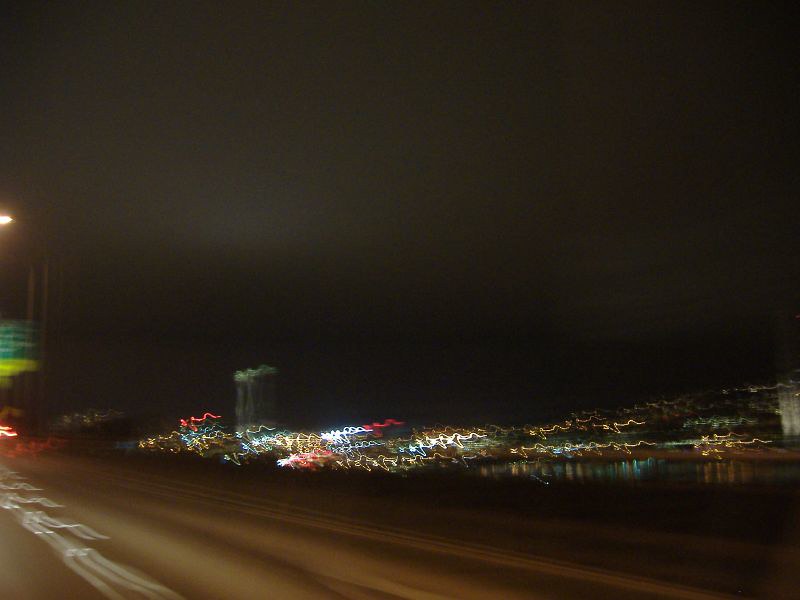The photograph appears to be taken from inside a moving vehicle, resulting in a significant blur and distortion across the image. In the bottom left corner, a roadway with white traffic lines is visible, indicating that the observer is traveling on this path. To the right of the roadway, a blurry nighttime city skyline is discernible, with various lights appearing as squiggly streaks due to the motion blur. In the bottom right corner, a hint of water is present, reflecting some of the distorted city lights. The rest of the background is enveloped in darkness, emphasizing the nighttime setting and contrasting with the illuminated and distorted skyline.